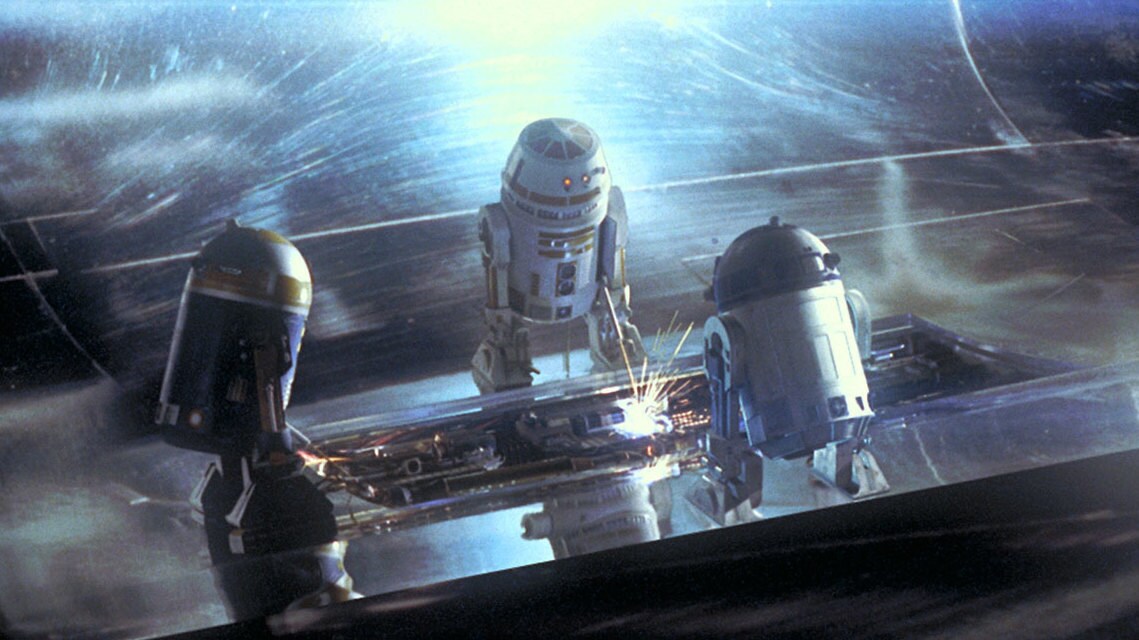The image is a vividly detailed scene from the 2005 movie "Revenge of the Sith," depicting three R2-D2-like robots working on the exterior of a spaceship. The background is illuminated with bright blue and white streaks, creating a striking contrast against the darker hues of the outer space setting. The central focal point is an open bay with exposed electronics, where the robots are engaged in repairs, emitting visible sparks from what appears to be a welding torch. Positioned strategically, one robot, identified as R2-D2, is located on the right side, while another similar bot with a distinct flat, conical section head is to the left. The third robot, also resembling R2-D2 but in a different color, completes the trio, all of whom are intently focused on their task. This detailed drawing, possibly a screenshot from the film, captures the intricate mechanics and the tense, pivotal moment where these droids, equipped with two arms, two legs, and expressive robotic eyes, navigate the dangers posed by pursuing fighters under the bright natural lighting of the scene.